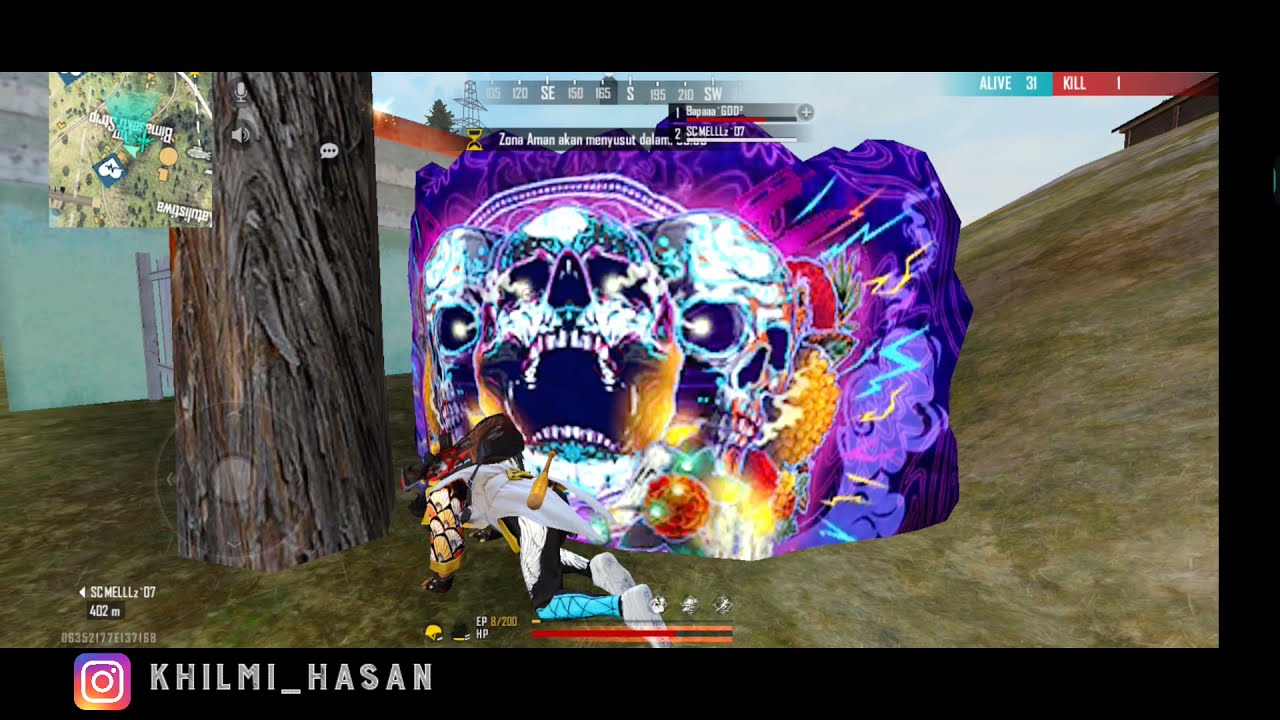The image is a detailed screenshot from a video game. The frame is horizontal and rectangular, surrounded by a consistent black border that is approximately an inch wide on all sides except the left-hand side, which features a thinner border. At the top of the image is a black rectangular strip encapsulating the scene. In the upper left-hand corner, a small map with white text indicates directions, while the upper right-hand corner displays the word "ALIVE" with the number 31 next to it, and "KILL" followed by the number 1.

The background features a light green concrete building and toward the foreground on the left side, there's a tree trunk sitting on a somewhat flat, medium greenish-brown ground that slopes upward to the right. 

Dominating the center of the image is a striking, jagged, and curvy purple square that appears to be an exploding square of light and energy. Three skulls sit prominently within this purple burst: one facing left, one facing right, and one facing forward. Each skull emits white light from their hollow black eyes, adding an otherworldly glow to the scene. Surrounding the skulls, colorful energy flows in shades of magenta, blue, yellow, green, and more purple, suggesting intense action or the aftermath of an explosion or impact.

At the bottom of the image, the text "kill me _Hassan" is visible, adding an additional layer of context to the scene. The overall composition indicates a dynamic moment in the game, possibly involving shooting, given the evident explosion and the term "KILL." The burst of colors and dramatic lighting highlight the frantic and vivid nature of this in-game moment.